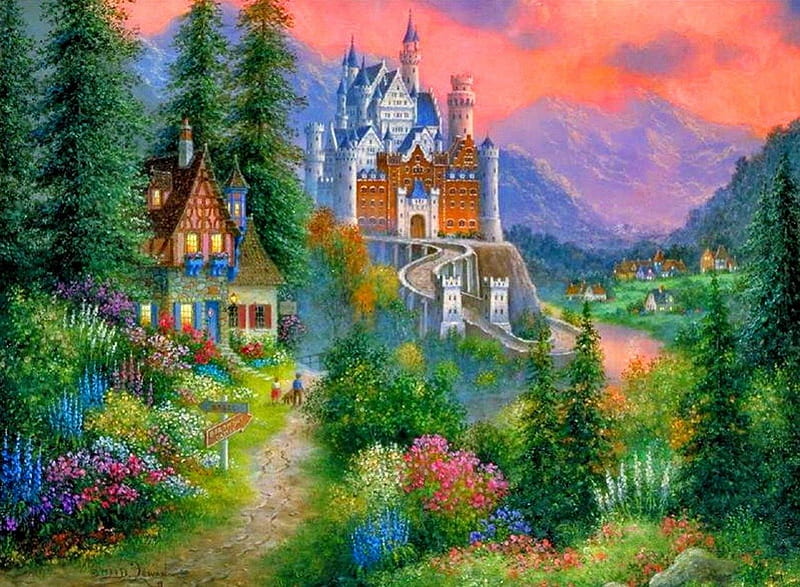This vibrant, painterly-style image depicts a whimsical, fairytale landscape under a striking red and pink sky. In the background, rugged purple mountains rise against the dusk-like horizon. At the heart of the scene stands a grand castle adorned with numerous turrets and spires, accentuated with blue roofs and brown walls. A winding road ascends to the castle, flanked by tall pine trees and vibrant flowers in a spectrum of colors—blues, purples, yellows, reds, and whites.

Nestled in the foreground to the left is a charming cottage with a brown roof, blue shutters, and flower boxes brimming with colorful blooms. The cottage glows warmly from its interior lights. A cobblestone path meanders past the cottage, where two children and a dog are seen walking, guided by a signpost directing them towards the castle.

To the distant right of the castle lies a quaint village of Tudor-style buildings with brown roofs, interspersed with green trees and fields. Above, the painterly sky swirls in shades of pink, red, and purple, creating a fantastical atmosphere. The overall composition, with its detailed flora, idyllic architecture, and enchanting lighting, brings to mind a scene from a fantastical storybook or an elaborate oil painting.